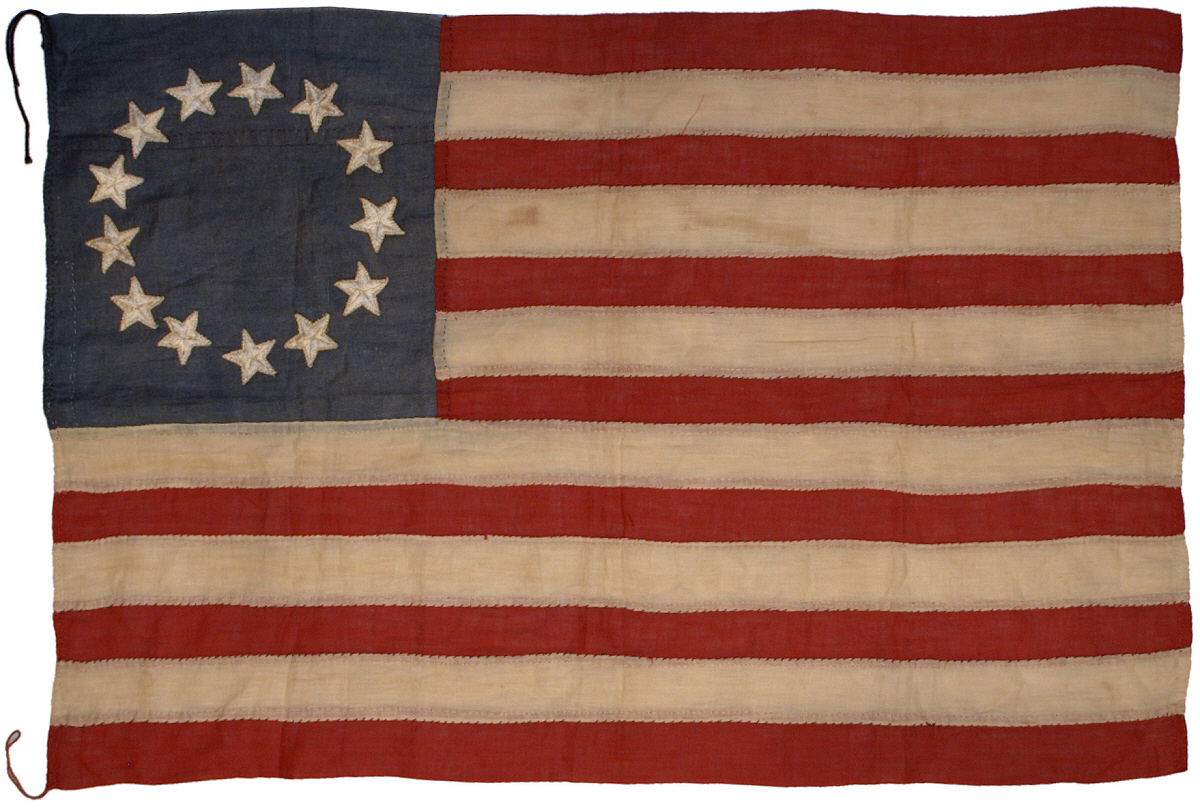This image depicts an antique American flag, specifically the historical Betsy Ross flag. The flag features 13 white stars arranged in a circle on a blue field located in the upper left corner, symbolizing the original 13 colonies. Additionally, it has 13 alternating red and white stripes, starting and ending with red, totaling seven red and six white stripes. The flag shows signs of aging, particularly on the white stripes, which appear worn and possibly artificially aged. Details such as visible stitching between the stripes and a few ties hanging off the left edge highlight its craftsmanship and vintage character. The overall appearance suggests it is made of a linen-like material and is in relatively good condition for its age.